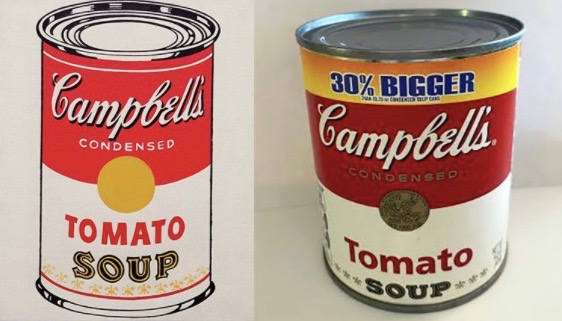The image depicts two cans of soup side by side. The can on the left features an animated design resembling a classic Campbell's soup label. This can has a silver top and a red upper half with "Campbell's Condensed" written in white letters. The lower half of the can is white and labeled "Tomato Soup" in red letters. At the center of the can, there's a yellow dot, with details including the letters 'CAMPBELL'S' rendered in white and "TOMATO" in red, while "SOUP" appears in black.

The can on the right is an actual photograph of a real can. It also has a silver top but includes a yellow banner near the top stating "30% Bigger" in blue letters. Below the banner, the label reads "Campbell's Condensed" with "Condensed" in brown letters. The lower portion of the label is dedicated to "Tomato Soup" written in red letters, with "SOUP" in gray. There is a brown circular emblem at the center of this can, featuring the iconic Campbell's design elements.